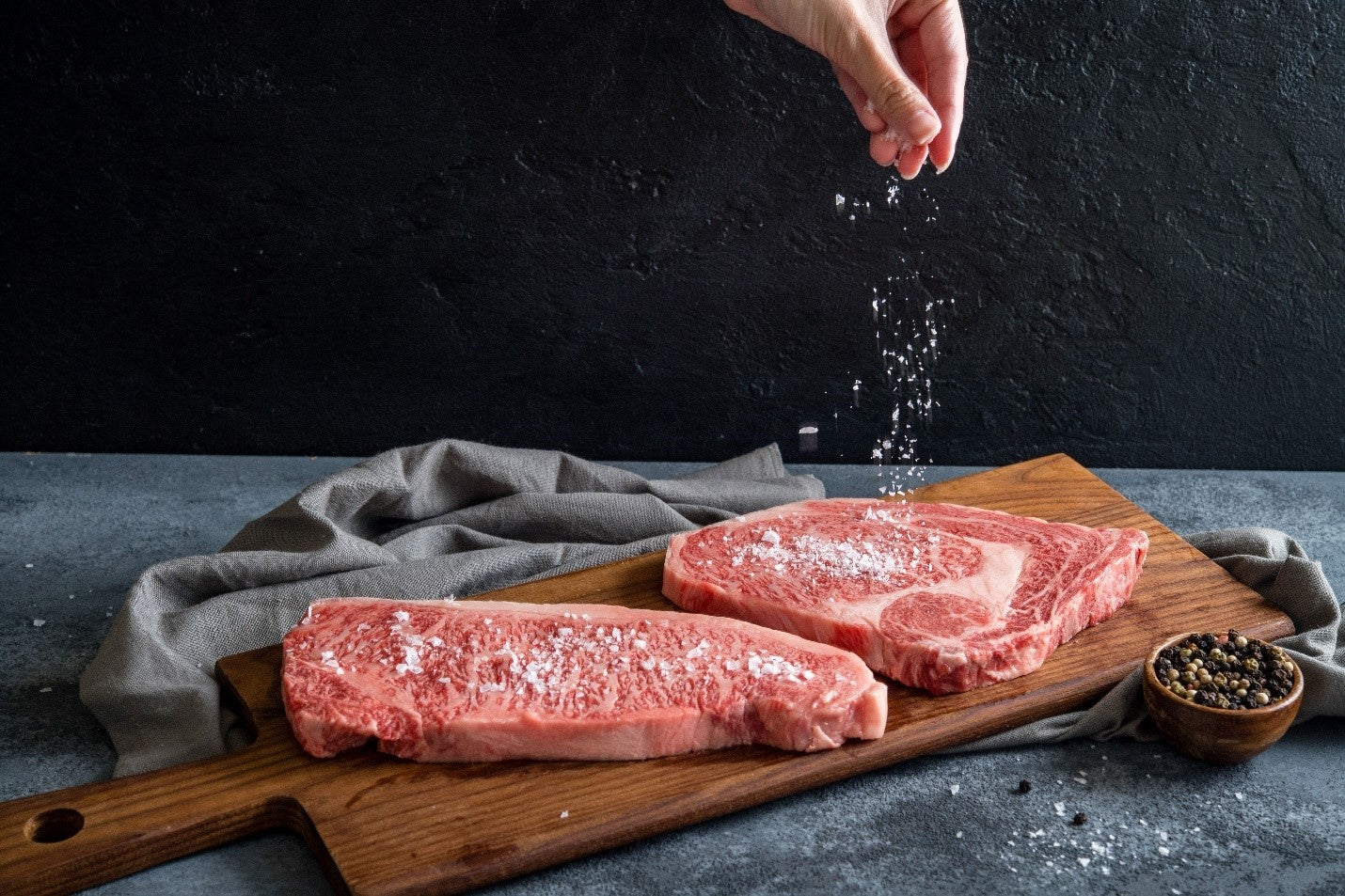In this elegant, eye-catching photograph, a person is captured mid-action, seasoning two large, reddish steaks on a medium-brown wooden cutting board with a handle and hole. The cutting board rests on a gray table in front of a stark black wall, highlighting the vivid colors of the raw meats. The person's fingertips are visibly sprinkling kosher salt onto a ribeye steak; the adjacent New York strip steak has already been salted. In front of the cutting board, a small wooden bowl filled with peppercorns and a folded gray napkin add to the scene's serene culinary atmosphere. The careful arrangement and contrasting background emphasize the steaks' freshness and luxurious quality, making this image a beautiful representation of the art of seasoning.